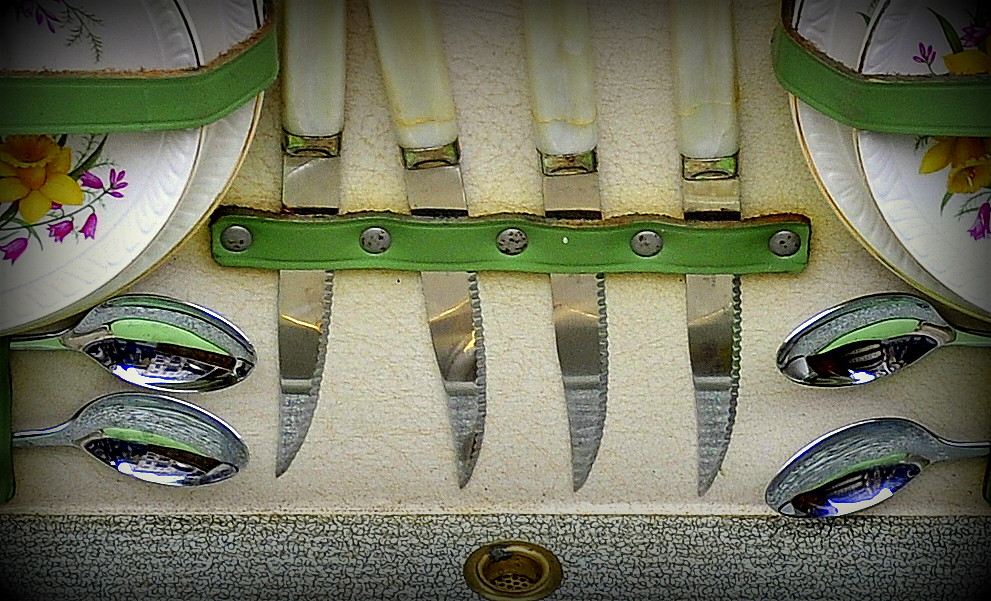This image showcases an elegant diningware set arranged meticulously within a box, focusing closely on the items. The central objects are four sharp steak knives with slightly serrated edges and smooth white handles accented with gold lines. These knives are aligned horizontally, held in place securely by a green leather strap featuring silver circular fasteners. Flanking the knives, on both the left and right sides, are pairs of large, clean, silver spoons arranged to mirror each other, with two spoons pointing inwards from each side. Surrounding the central cutlery, there are white china plates adorned with vibrant floral patterns, including yellow and purple flowers and green foliage. Each stack comprises two plates, highlighted with golden rims, and they are also held in place by green leather straps. The overall backdrop features a light-colored placemat with a subtle cobblestone design in gray and white, adding to the sophisticated presentation of this well-organized dining set.